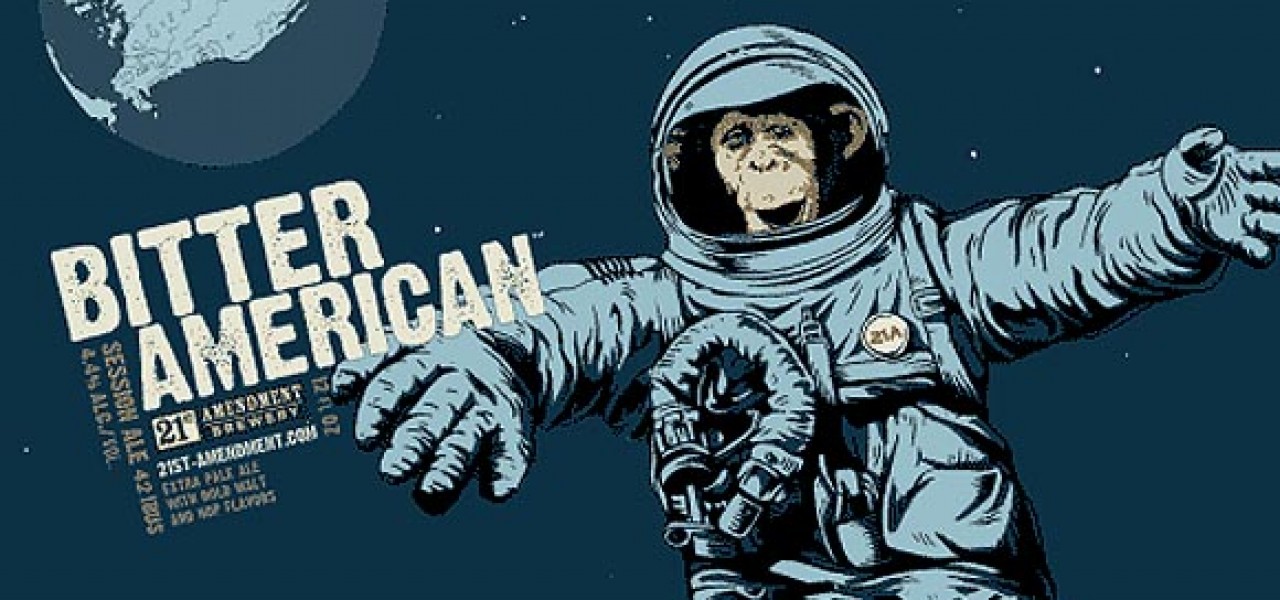This image is a vintage-style advertisement poster for "Bitter American Session Ale" by the 21st Amendment Brewery. Dominating the right side of the poster is a chimpanzee dressed in a spacesuit, floating in space with arms extended and mouth open in what appears to be laughter. The spacesuit features a beige badge that reads "ZIA". The background is a dark turquoise, representing outer space, punctuated by white dots symbolizing stars. Planet Earth is visible in the upper left corner. Large white text on the left side of the poster reads "Bitter American", followed by smaller, somewhat unclear text that includes "Session Ale 4.2 IBUs 4.4 ALC". Additional text below reads "21st Amendment Brewery" and a website URL, "21stamendment.com". The entire design uses a limited color palette of blues, black, and white.